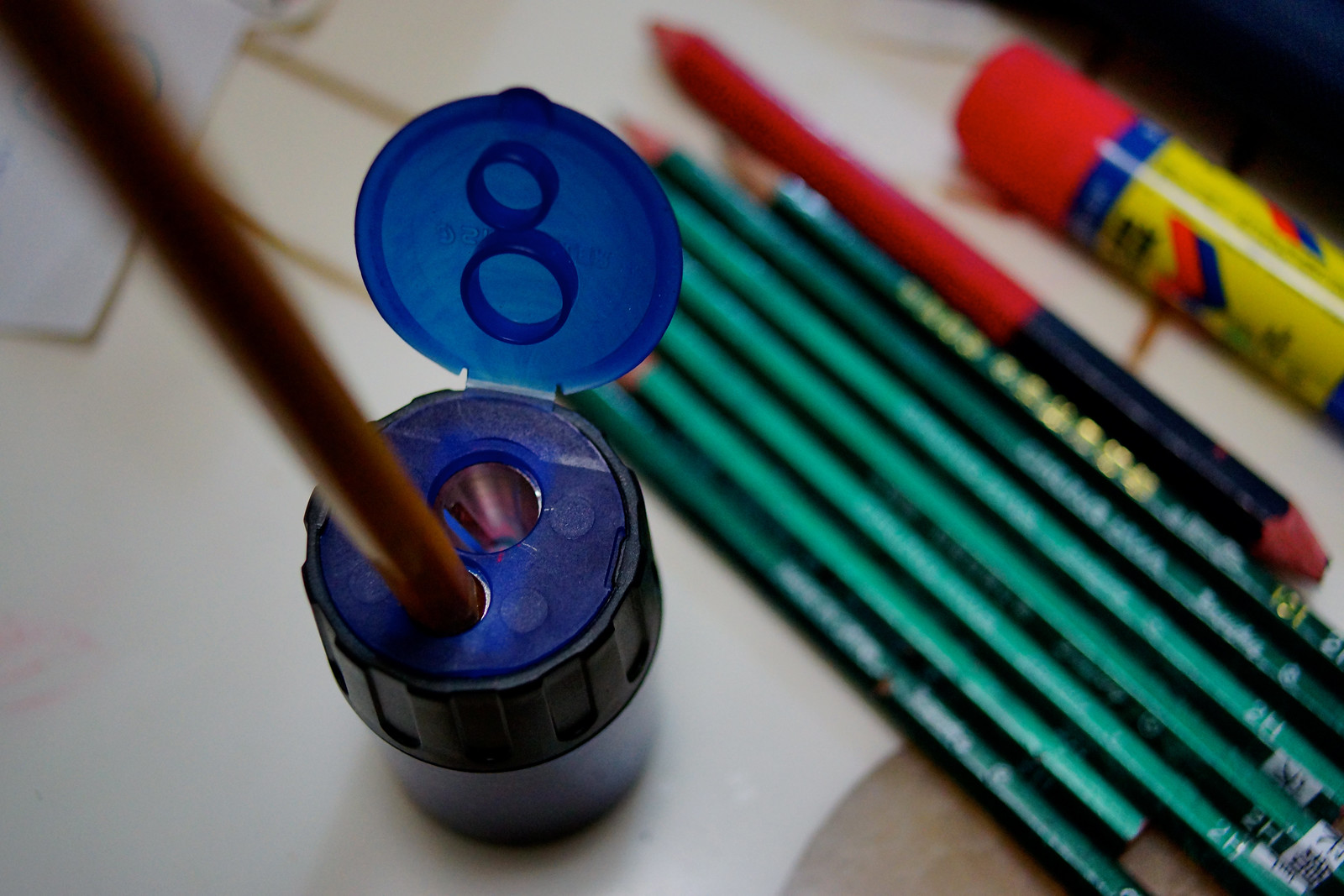The photograph showcases a blue cylindrical pencil sharpener prominently in focus, positioned on a white piece of paper atop a wooden table. The sharpener, with its lid flipped open, reveals two holes: a larger one for thick pencils and a smaller one for thin pencils, with a pencil currently inserted and being sharpened in the smaller hole. The sharpener's design includes a black ribbed ring for grip and a repository underneath the lid to collect shavings. The background, slightly blurred, features an array of seven green pencils and a thick, double-headed pencil colored red and black, all arranged diagonally from the bottom left to the top right of the image. Additionally, a glue stick with a red cap and a predominantly yellow body is situated to the right of the pencils, adding a splash of color to the scene.